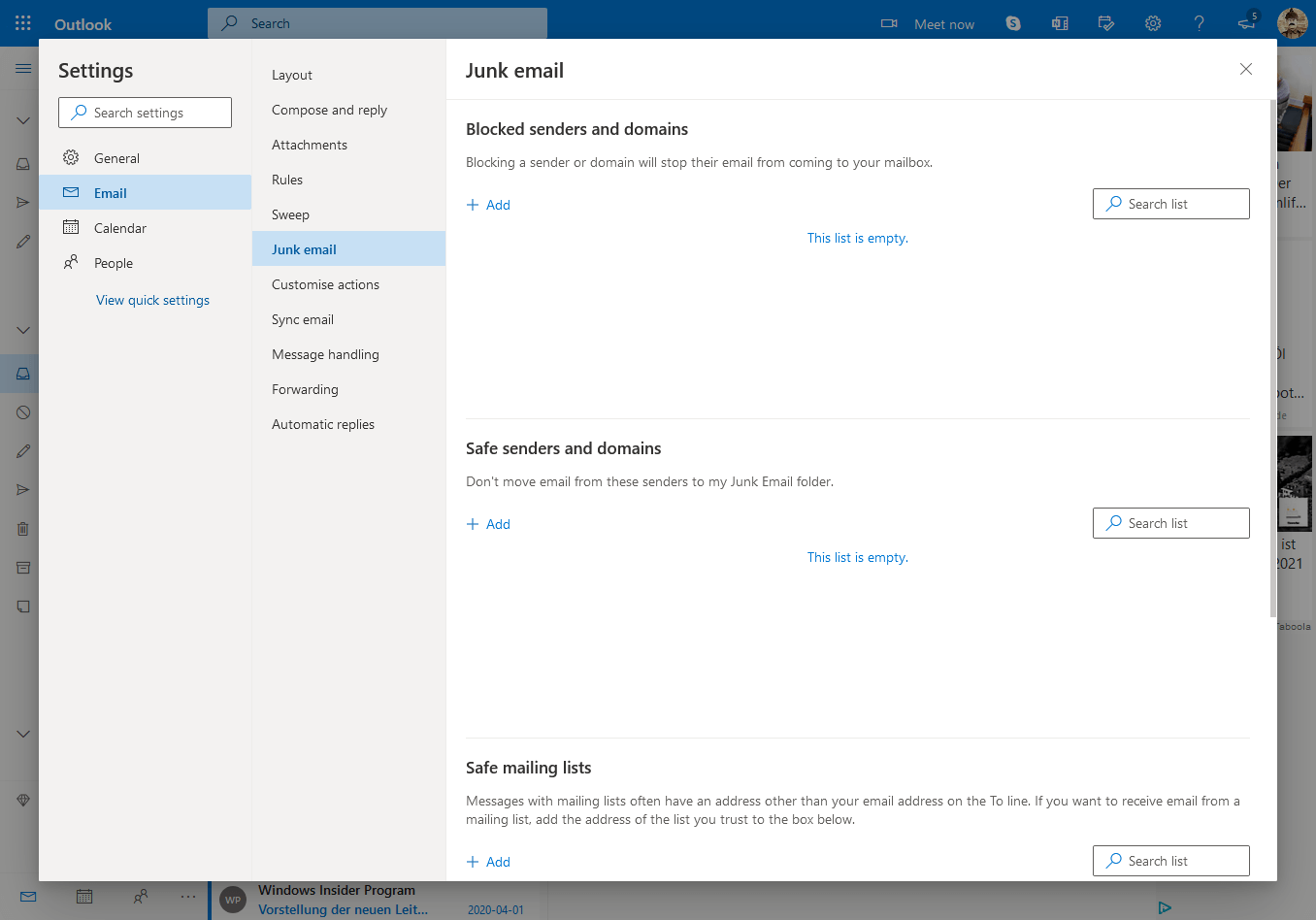Here is a detailed and cleaned-up caption for the image:

---

This screenshot captures the Settings page of the Outlook Windows application. At the center, framed by a white box, is the Settings dialog box providing a range of customization options. The left-hand side of this dialog box features a vertical tab list, including categories such as General, Email, Calendar, and People. The 'Email' tab is highlighted in blue, indicating it is currently active. Adjacent to this, another sub-option, 'Junk Email,' is also highlighted in blue text, showing it as the selected setting to edit.

On the right-hand side of the box, the top header reads 'Junk Email' in black text. Here, users can manage their junk mail settings, featuring options for 'Blocked senders and domains,' 'Safe senders and domains,' and 'Safe mailing lists.' This section allows users to configure their email filters by blocking unwanted emails and domains that will be automatically directed to the junk folder. Conversely, users can whitelist specific emails to prevent them from being marked as junk, ensuring important messages are delivered to the primary inbox.

Surrounding the settings dialog box, the broader Outlook application is visible against a dark-themed interface. The top left corner displays 'Outlook' in white text over a blue bar, providing branding and context. In the top right corner, several functional icons are present, including a gear symbol for accessing the Settings page, a white question mark for the Help page, and a profile picture icon for opening and editing the profile settings.

---

This detailed caption captures all the elements and functionalities visible in the screenshot clearly and concisely.